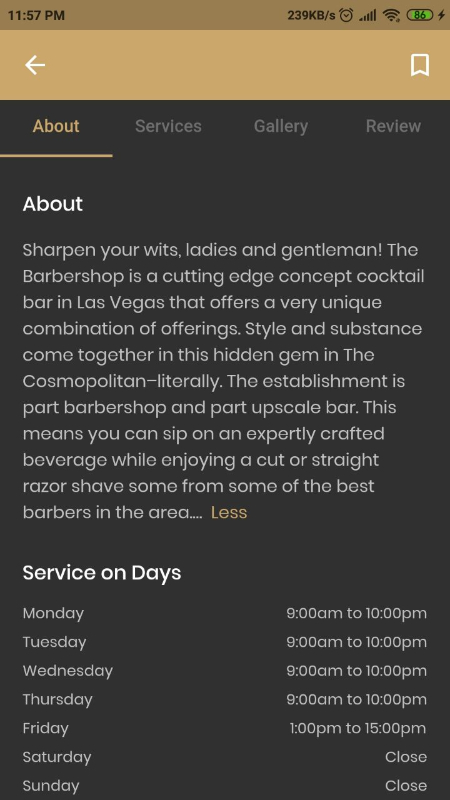This is a detailed photograph showcasing the business information of a mobile app interface for a barbershop and cocktail bar in Las Vegas. At the top of the screen, there is a beige header featuring a white arrow pointing to the left and a white bookmark symbol on the right. Directly below the header, there are four evenly spaced options: "About," "Services," "Gallery," and "Review." The "About" option is highlighted in beige with a matching underline, while the others are in dark gray text.

Below these options, set against a dark gray background, the heading "About" appears in white text. In the subsequent paragraph of white text, the app provides an intriguing description: "Sharpen your wits, ladies and gentlemen. The Barbershop is a cutting-edge concept cocktail bar in Las Vegas that offers a very unique combination of offerings. Style and substance come together in this hidden gem in the Cosmopolitan, literally. The establishment is part barbershop and part upscale bar. This means you can sip on an expertly crafted beverage while enjoying a cut or straight razor shave from some of the best barbers in the area..." Next to this paragraph, there is a beige "less" indicator for collapsing the text.

Further down, a bold white text heading labeled "Service Hours" is followed by a detailed list of operational days and times in smaller white text. The hours are listed as follows:
- Monday: 9 am to 10 pm
- Tuesday: 9 am to 10 pm
- Wednesday: 9 am to 10 pm
- Thursday: 9 am to 10 pm
- Friday: 1 pm to 3 pm
- Saturday: Closed
- Sunday: Closed